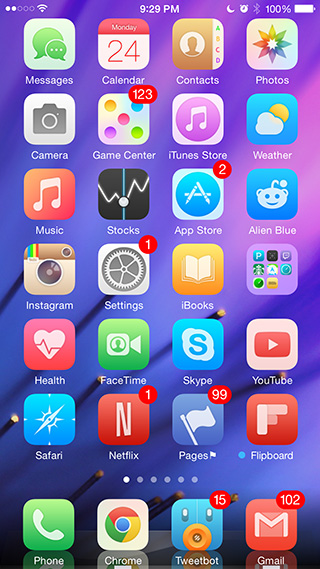A screenshot is shown displaying an antiquated phone menu, suggesting it could be from either an iPhone or an Android device. The interface exhibits an old design style, showcasing various apps available for selection. The background is a vibrant mix of dark blue and light purple colors. In the top left corner, the Wi-Fi signal and service bar indicators are visibly present. Centrally positioned at the top of the screen is the current time, and in the upper right corner, icons for Bluetooth, battery status, and an active alarm are displayed.

The main section of the screenshot reveals a scrollable menu with multiple app icons. At the very bottom of the screen, four frequently used app icons are positioned from left to right: Phone, Chrome, Tweetbot, and Gmail. The Phone app icon is depicted as a green box with a white phone symbol. The Chrome icon is a multicolored sphere featuring red, green, and yellow with a blue circle in the center. The Tweetbot icon, representing a now-defunct app, is an illustration of a robotic bird, possibly inspired by Tweety Bird, meant for interacting with Twitter. Finally, the Gmail icon is characterized by a red box with a white and red 'M' in the middle.

Overall, the screenshot encapsulates a nostalgic view of an older mobile device interface, enhanced by a colorful and slightly dated design.